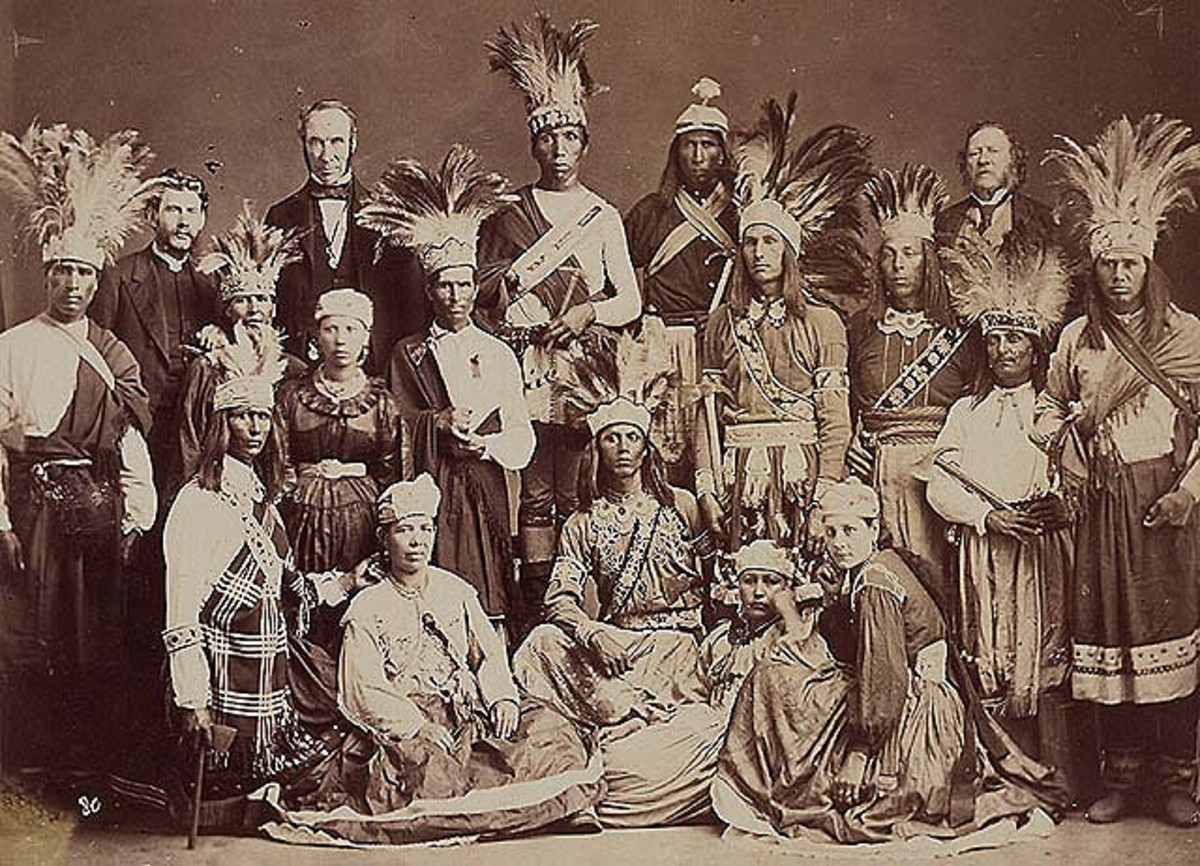The image is a landscape-format, black-and-white photograph that appears to be from the late 19th century. It features a group portrait with around a dozen Native individuals and three Western men, who seem to be either English, American, or European. The Native people are dressed in traditional attire, adorned with feathered headdresses that vary in size between men and women. The women seem to be wearing smaller hats without feathers. The Western men are dressed in formal suits. The group stands solemnly, looking directly at the camera. The photograph captures a stark contrast between the traditional native outfits, resembling dress-like robes, and the formal Western suits, highlighting the cultural differences between the two groups.